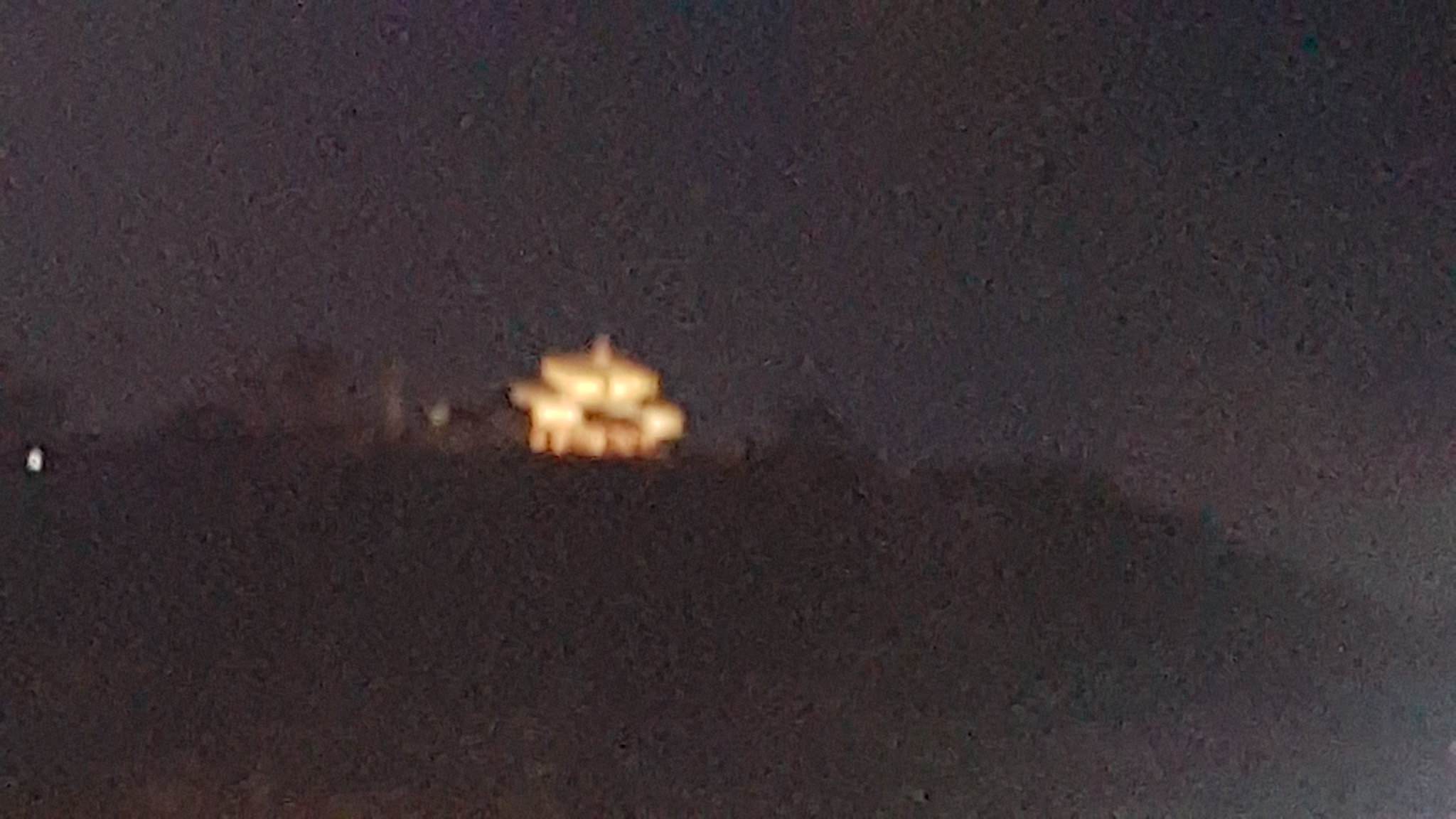This is an extremely dark, blurry, and pixelated image, reminiscent of an old photograph taken with a low-quality, old-fashioned camera. The photo, captured at night, centrally features a faintly lit structure that appears slightly left of center and resembles a building. The building seems to sit atop a hillside or a mountain, which is silhouetted against an almost black sky. The hillside takes up roughly half the height of the image from the bottom, and the grainy quality makes it difficult to discern any specific details. There are no visible markings, people, animals, vehicles, or motorized structures within the image, which is wider than it is tall. Due to the overwhelming darkness and poor focus, the photograph resembles the effect seen when zoomed in excessively, rendering most elements indiscernible.